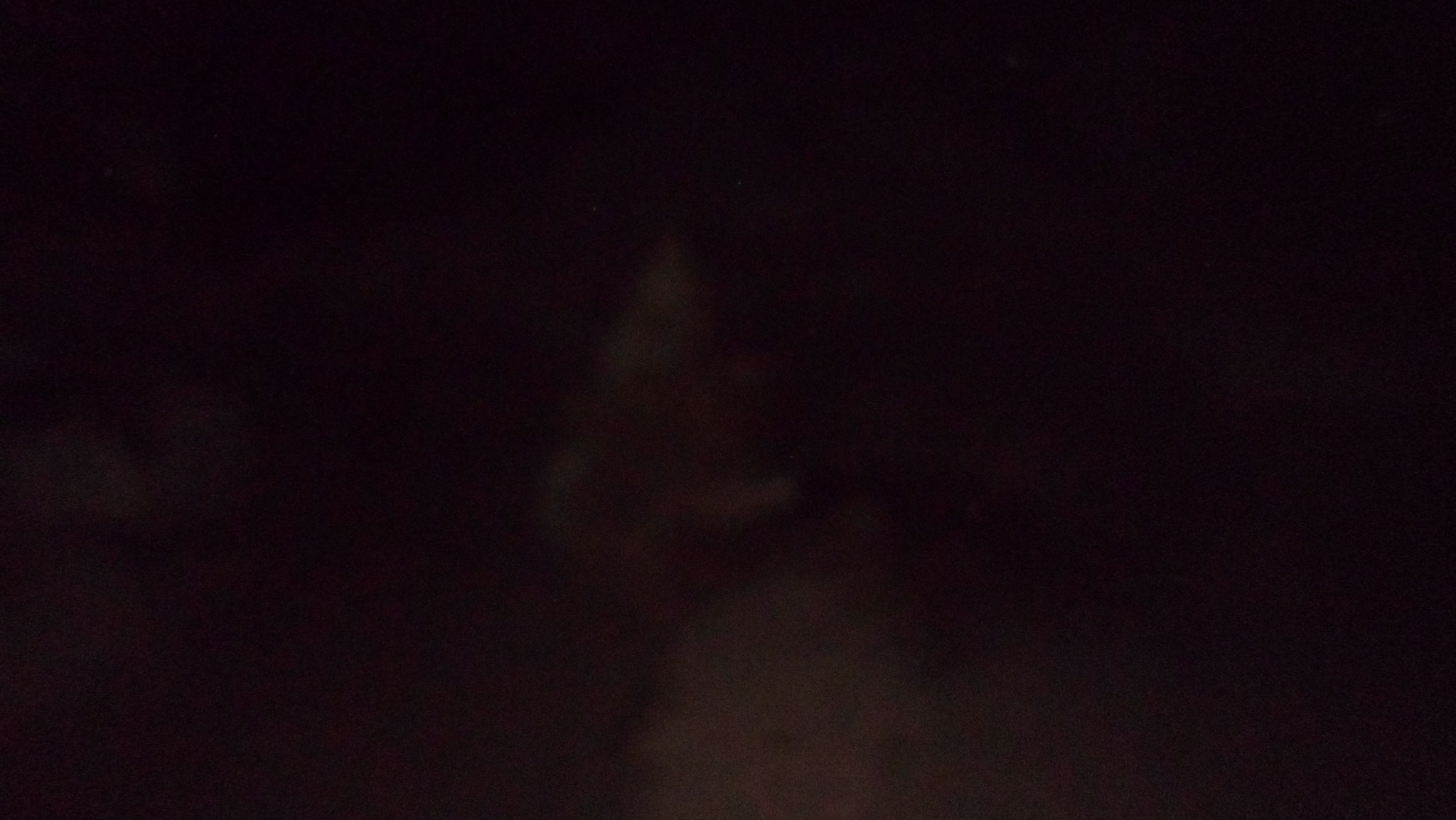The image appears, at first glance, to be entirely black, suggesting it might be an error or a photograph taken in extremely low light. On closer examination, subtle details emerge in the dark and grainy background. Faint, wispy triangular shapes and a grayish blob can be seen towards the center and far left of the image. Upon even closer scrutiny with minimized lighting, the left side of a woman's face becomes barely perceptible, seemingly captured from a rear three-quarter view. The contours of her ear, cheek, hairline, and a hint of her neck are faintly visible, suggesting that some light fell on her as she looked slightly upwards. The overall lack of clarity and absence of text further contribute to the enigmatic and indistinct nature of this very dim and blurred photograph.